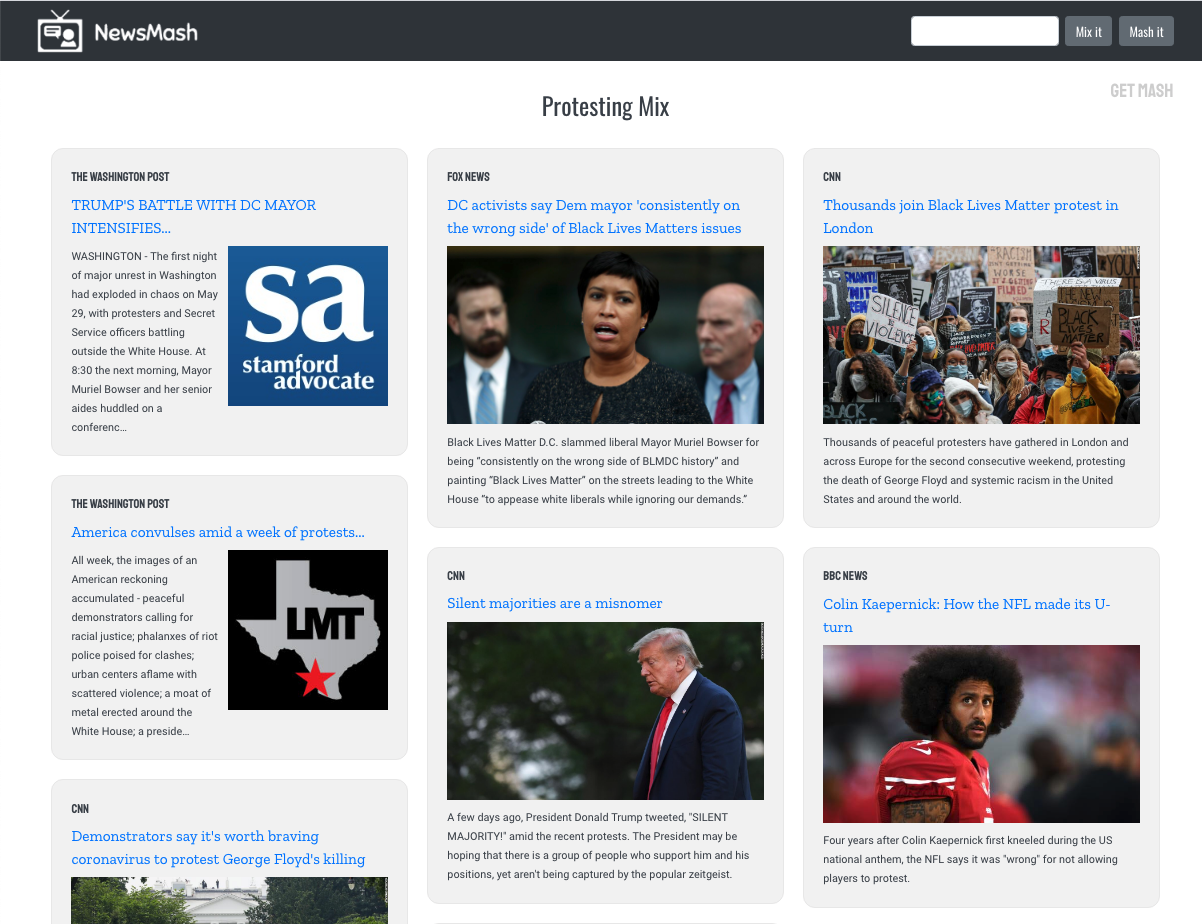A screenshot of the News Mash website, featuring a sleek black header with a TV icon next to the site's name, "News Mash." The header also contains a white rectangular section on the right with two clickable buttons labeled "Mix It" and "Mash It." Below the header, the main content area displays six news article previews arranged in two rows of three, with an additional partially visible article on the far left.

**Top Row:**
1. **Trump's Battle with D.C. Mayor Intensifies** - An article from Fox News highlighting claims by D.C. activists that the Mayor consistently opposes Black Lives Matter issues.
2. **Thousands Join Black Lives Matter Protest in London** - A report on the significant turnout for a Black Lives Matter protest in London.

**Bottom Row:**
The details for the bottom three articles and the cut-off article on the far left are not fully visible in the screenshot.

There is a snippet of a conversation overlay, indicating the image was likely shared during a discussion or presentation: 
"Tori in the house. Why don't you put him in the truck? No, she's going to die of heat stroke. I'm going to get air conditioning on. You're probably loving that you're doing this. Oh yeah, I am."